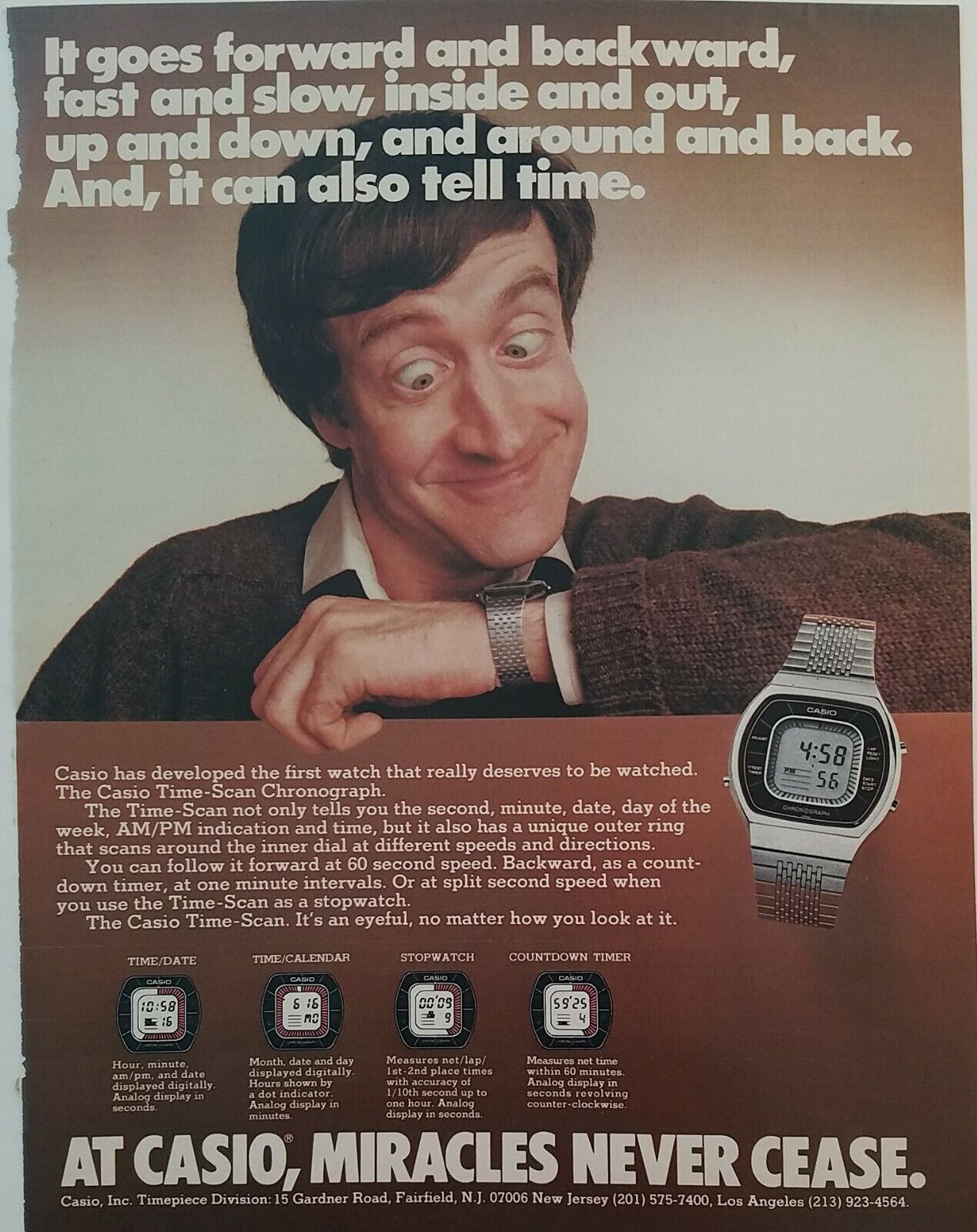This vintage advertisement, likely from the 1980s, features a white man with dark brown hair wearing a brown jacket over a white shirt. He stands centrally in the image, cross-eyed as he gazes intently at the silver digital watch on his wrist, which adds an element of humor and curiosity. The backdrop is a simple brown wall or table, creating a rustic context for the modern gadget. 

The watch he's showcasing has a sleek silver band and casing, with a black ring inside the dial bearing the name "Casio" and the slogan "miracles never cease" inscribed at the bottom. The digital face displays various times such as 4:58, 5:56, while separate images show 10:58, 6:16, 00:09, and 5:24, highlighting its multi-functional capabilities. 

Text on the ad describes the Casio Time Scan Chronograph in detail, emphasizing its ability to display seconds, minutes, days, dates, and A.M./P.M. indicators. It boasts a unique outer ring that moves at different speeds and directions—forward at 60-second intervals, backward as a countdown timer, and even at split-second speeds for stopwatch functions. The description showcases the watch as a marvel of innovation, declaring it the first watch "that really deserves to be watched." Additional paragraphs break down its time, calendar, stopwatch, and countdown timer functions, reinforcing Casio's tagline that "miracles never cease."